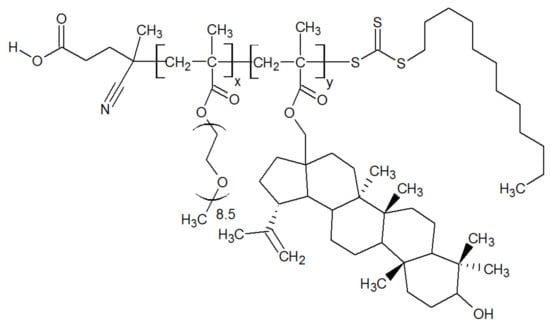This image depicts a detailed chemical chart on a white background with black text, primarily used to illustrate the formation and breakdown of copolymers in a classroom setting. At the top, the diagram starts with letters 'H' and 'O' connected horizontally by a line, followed by a vertical jagged line descending. Continuing horizontally, we encounter chemical symbols like 'N' connected to 'CH3' via a long line, and several 'CH2' groups connected by smaller lines. To the right, there are distinctive segments where 'S' appears repeatedly in a vertical alignment, leading towards a horizontally terminating 'H3C'. The structure also includes octagonal and rhomboidal shapes near the bottom marked with 'CH3' and 'OH'. Additionally, the molecule features curves, double bonds of oxygen and sulfur, and various notations such as brackets and parentheses indicating attached groups. Triangles, both solid and outlined, are also part of the intricate display of molecular topology.